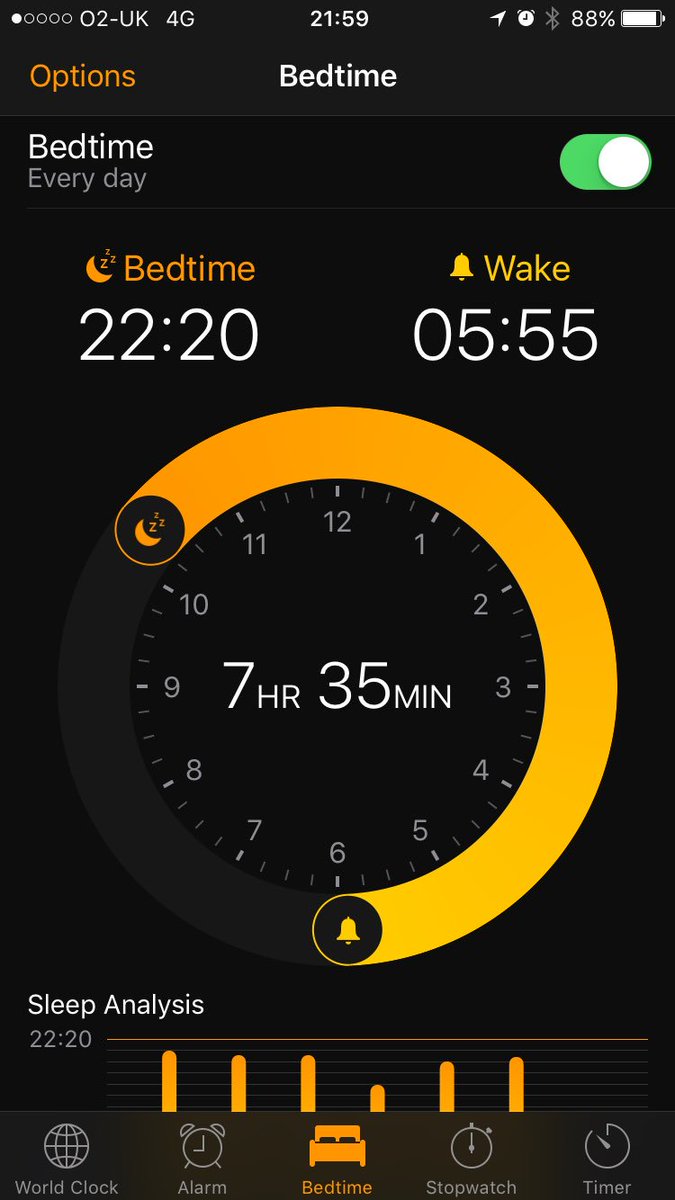The image showcases the Bedtime feature in the Clock app on an iPhone, displayed in Dark Mode. The primary background color is black, while the header features a gradient from dark gray on the left. The header contains the word "Options" in an orange, sans-serif font, and "Bedtime" in bold, white font.

Just below the header, there's a rectangular section with a black background. In the upper-left corner of this section, it says "Bedtime" in white text, with "Every day" in smaller, gray font beneath it. To the right, a green toggle switch indicates that the feature is activated; the switch has a white circle on the right side.

Lower down, there's a crescent moon icon with its top tip pointing to the upper left and the bottom tip to the lower right, accompanied by orange Z's. To the right of this, "Bedtime" is written in large, white font. Below this, in even larger white font, it reads "22:20" (10:20 PM). Adjacent to this, a yellow bell icon signifies the wake-up time, with "Wake" written underneath it in large white letters. The wake-up time, "05:55" (5:55 AM), is prominently displayed below.

In the lower part of the screen, a large clock is visible, featuring an ombre design that transitions from orange at 10 o'clock to yellow at 6 o'clock. At the center, "7 H R 35 M I N" is displayed in large white letters, indicating the total sleep duration.